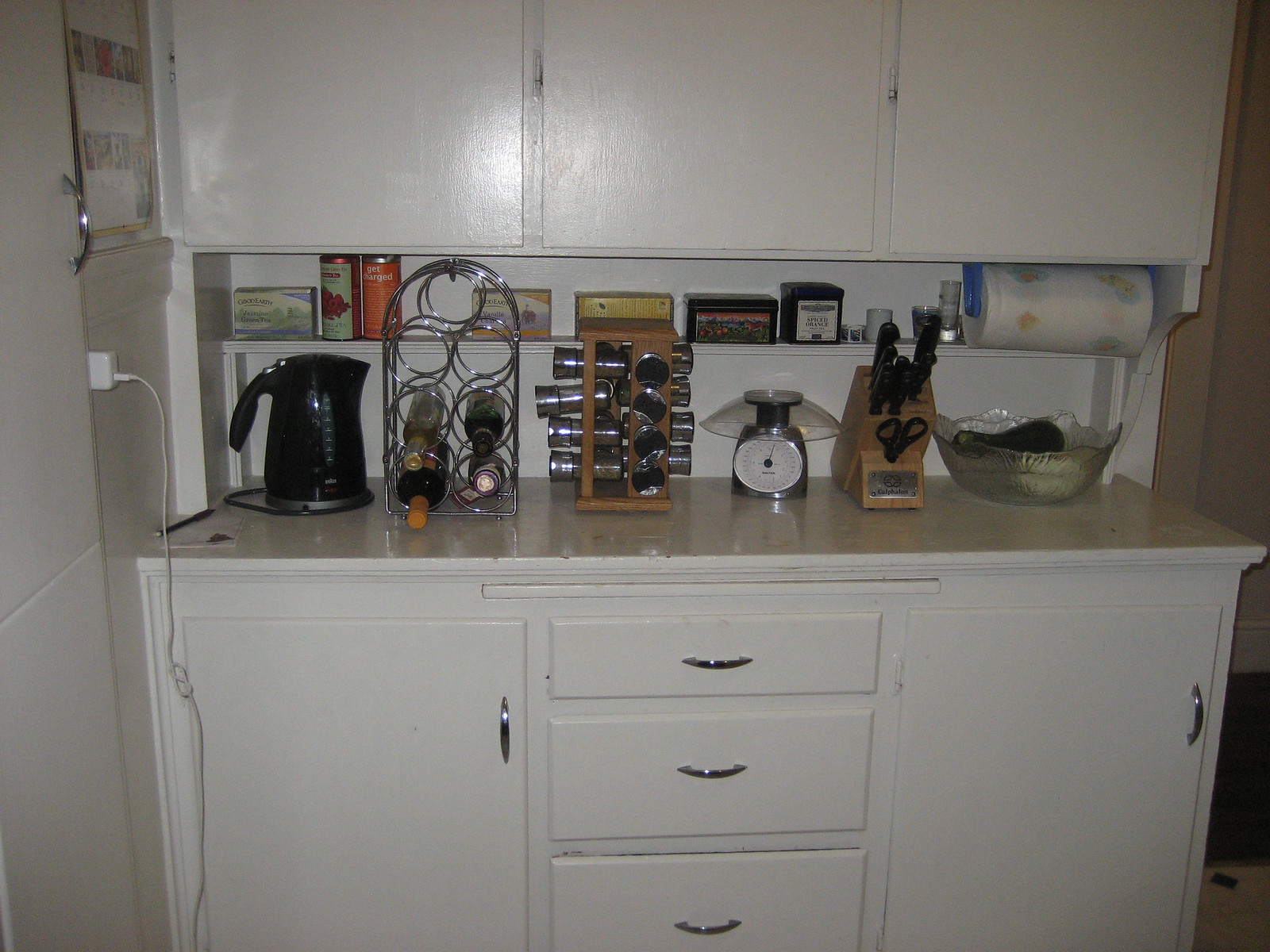The photo captures a well-organized kitchen countertop devoid of a sink, maintaining a clutter-free appearance. Central to the scene is a variety of kitchen essentials neatly arranged. On the left, a large pouring cup stands next to a collection of wine bottles nestled in a wine rack. The central section of the counter features a spice rack and a kitchen scale, with a wooden rack holding various knives and scissors beside it. A glass bowl containing an unknown item also rests on the counter.

Above the counter, a shelf stocked with paper towels and several tin cans is installed, adding to the kitchen's functional storage. At the top, white cabinet doors provide additional storage space, complementing the matching cabinetry below the counter, which includes drawers with visible handles. To the left, a white phone charger is plugged into an outlet, indicating the convenient charging setup on this side of the counter. Finally, another white cabinet is positioned nearby on the left, adding to the kitchen's cohesive and practical design.